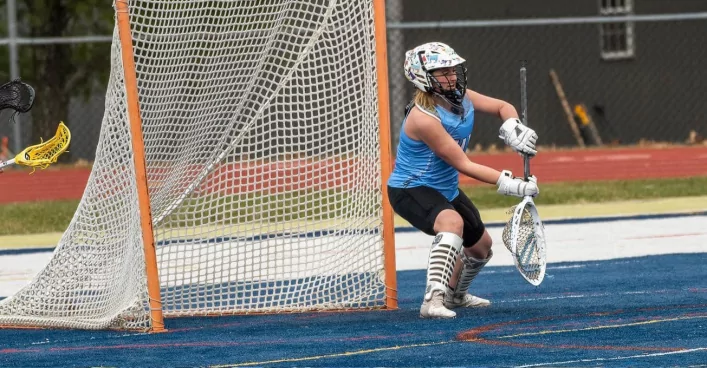In this detailed photograph of a lacrosse game, a woman stands focused in front of a moderately-sized goal with a white net and orange crossbar, which is smaller than a soccer net but larger than a hockey net. She is equipped as a goalkeeper, wearing a white helmet with a black metal cage, thick white gloves, shin guards, black shorts, and a blue jersey. She clasps a large racket with a net, resembling a shallow fishing or bug-catching net, which contrasts with the more slender rackets seen on the left side of the image. Her short blonde hair peeks out from under her helmet, and her stance indicates she is ready to intercept the ball. The field is distinctly blue, possibly blue astroturf, with painted markings, while the background includes a corrugated metal shed, brick lining, a garden, and a running track. The combination of her protective gear and concentrated expression highlights the intensity and anticipation of the game.